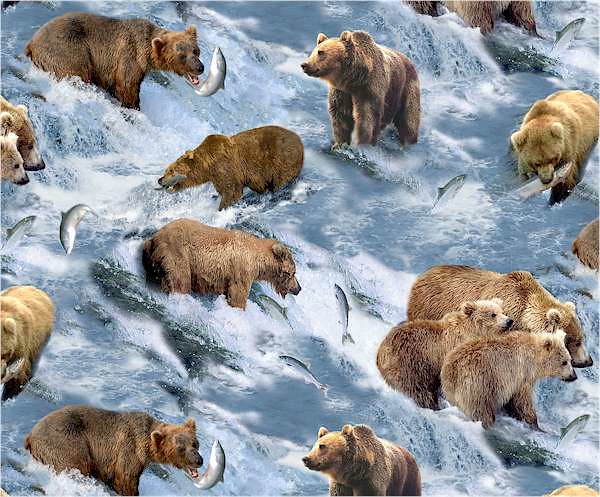This vibrant, detailed illustration depicts a dynamic scene of grizzly bears engaged in a lively salmon hunt within a rushing, white-water river. The river, characterized by cascading rapids and white water, gives a vivid sense of turbulent motion as it flows over submerged stones, creating varying levels and eddies. In the midst of this powerful flow, approximately eight to ten grizzly bears of varying sizes and colors, ranging from dark brown to pale brown, are scattered across the river. Some bears are standing on rocks, while others have their heads submerged, eagerly hunting for salmon. The air is filled with the splashing of salmon, about nine in total, leaping out of the water in a desperate bid to escape. One bear on the right triumphantly holds a gleaming fish in its jaws. This compelling illustration captures the energy and tension of these magnificent creatures amidst the swirling waters in their relentless pursuit of a meal.